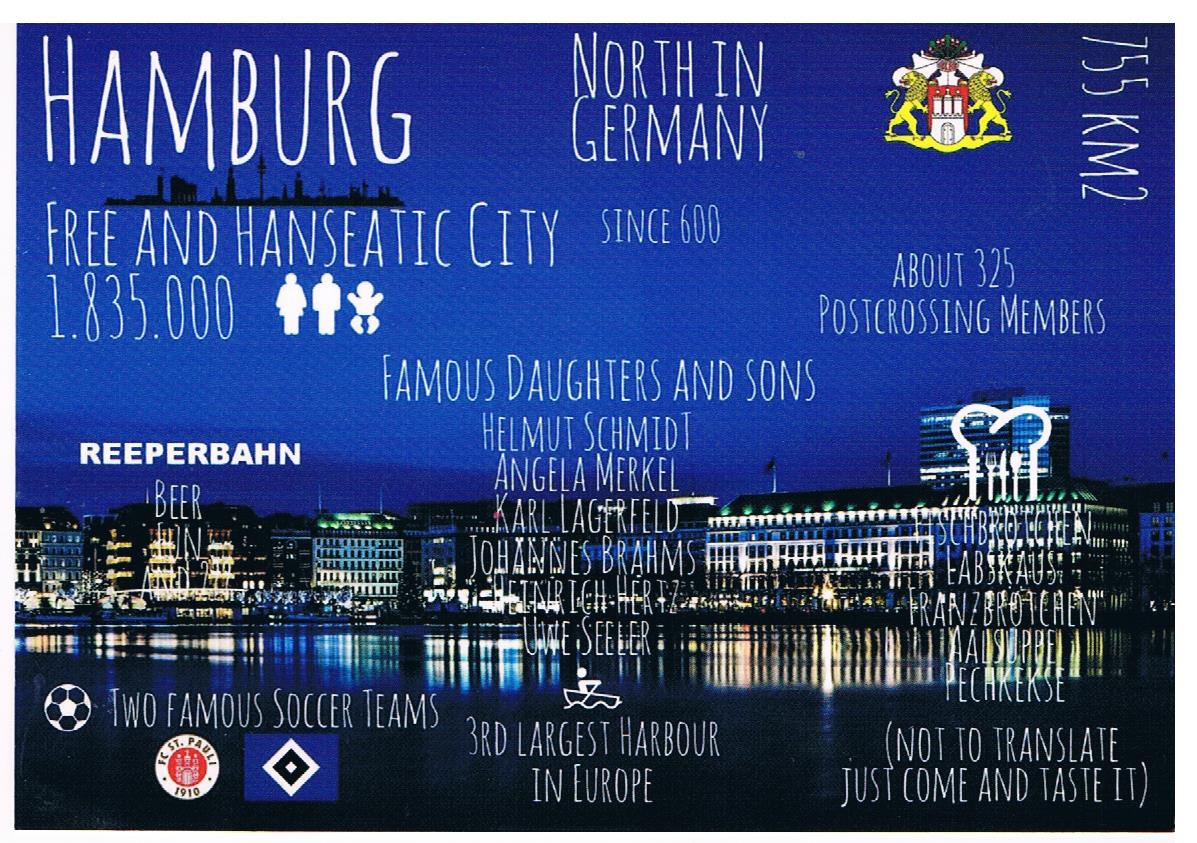The advertisement for a major event in Hamburg, Germany, features a detailed night-time view of the Hamburg skyline across a large body of water. The upper left corner prominently displays "Hamburg" in white text over a dark and darker blue background. Below it, in black text, it reads "Free and Hanseatic City, 1.835.000" along with a depiction of a man, woman, and child in silhouette. The middle top section features the phrase "North in Germany" in white, accompanied by a yellow and red symbol nearby. Underneath this, in white, it states "Since 1600, about 325 post-crossing members." Centered on the image is the phrase "Famous Daughters and Sons" followed by a list of six names. The picturesque night-time harbor scene is further emphasized with descriptions such as "Third largest harbor in Europe" in the bottom center and additional text in the far right lower corner, "Not to translate, just come and taste it." The left side references "Two Famous Soccer Teams" with a soccer ball icon and logos of two soccer clubs, one with a white circular design and a red interior, and the other with a blue flag shape and a black and white diamond. Above some buildings on the left is the text "Reeperbahn Beer," and atop a building on the right is an image of a chef's hat with utensils inside. The entire advertisement is characterized by its numerous white text elements set against the dark, illuminated backdrop of Hamburg's waterfront.